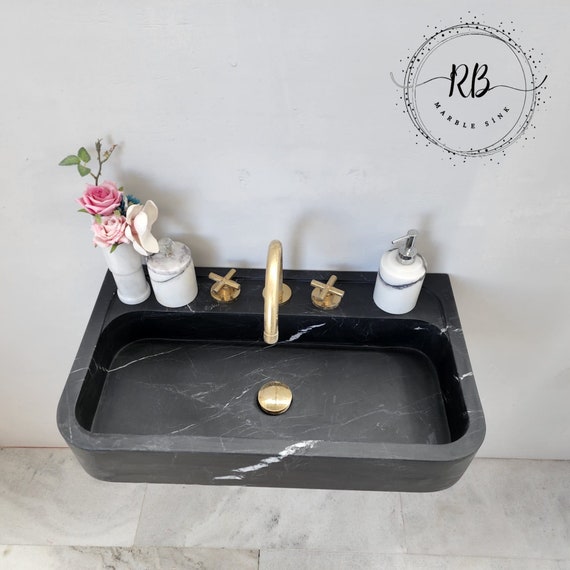The advertisement showcases a sleek, modern rectangular black marble sink, elegantly contrasted with retro-styled bronze or gold fixtures. Prominently displayed within a pristine bathroom setting, this floating sink stands against a bright white wall and is complemented by a white and gray marble tiled floor. The opulent black sink features subtle white streaks, enhancing its luxurious appeal. Accentuating this stylish setup, a white soap dispenser, a vase with pink and light pink flowers, and another white marble-patterned dispenser are thoughtfully arranged on the sink's surface. In the top right corner of the image, the detailed and sophisticated logo of RB Marble Sink adds a finishing touch, encapsulating the brand's blend of modernity and classic charm.